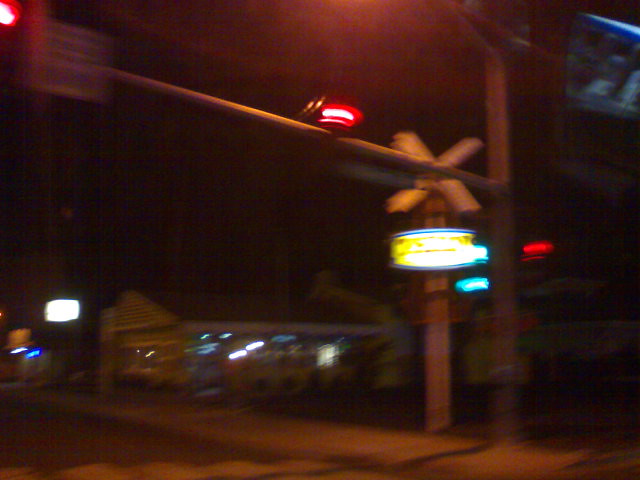In this nighttime photograph, the image appears blurry, obscuring some details but still providing context. The focal point is an outdoor setting featuring a square. In the background, a building stands illuminated, showcasing lights and a distinctive white triangular peak atop a flat brown roof. This building might be a restaurant, though it's difficult to ascertain. Nearby, a sidewalk runs parallel to the structure. A train crossing is indicated by visible signage, including a prominent white "X" and a red traffic light, presumably for the approaching train. An illuminated yellow sign with blue trim is present, though its exact purpose is unclear due to the light’s glare.